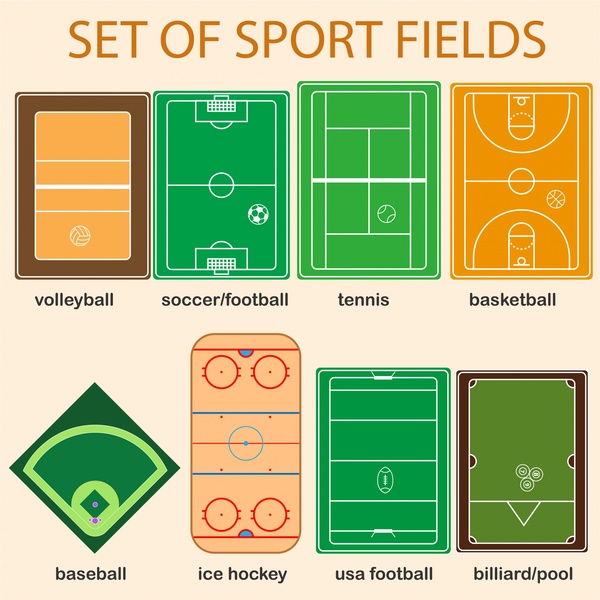This image presents a digitally created diagram set against a light tan or pinkish background, showcasing different sports fields arranged for an informational presentation. At the top of the image, bold capital letters read "SET OF SPORTS FIELDS." Below this heading, the diagram is divided into two rows, each containing four fields. The top row features smaller diagrams of volleyball, soccer/football, tennis, and basketball fields, each labeled in black lettering below their respective images. The bottom row includes diagrams for baseball, ice hockey, USA football, and billiards/pool, similarly labeled.

The fields are depicted in varying colors including tan, green, light green, orange, brown, dark brown, red, blue, yellow, white, peach, and black. The positioning of the diagrams is structured and well-organized, with each field placed adjacent to the next, creating a neat and cohesive layout. This setup is ideal for a presentation, providing a clear and detailed visual guide to various sports fields.